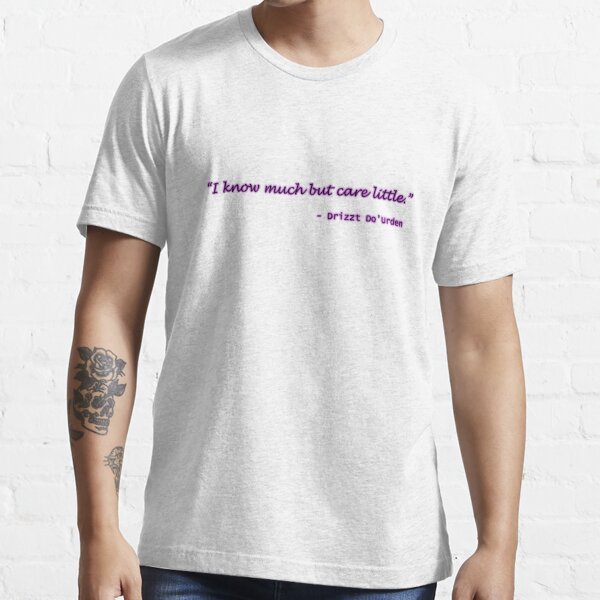The image showcases a man standing against a white painted brick wall, captured from his neck down to his waist. He is wearing a heathered white crewneck t-shirt adorned with purple script that reads, "I know much, but care little," followed by the attributed name "Drizzt Do'Urden." The man's skin is of a lighter complexion. On his right forearm, he has a detailed tattoo featuring a flower emerging from a skull, primarily inked in dark green. There is another tattoo visible near his wrist, though its details are obscured due to the arm's positioning. His hands rest at his sides, and the bottom hem of his blue jeans is barely visible at the lower edge of the image. The bright lighting highlights the clean and clear details of the scene, though it is not clear if the location is indoors or outdoors.